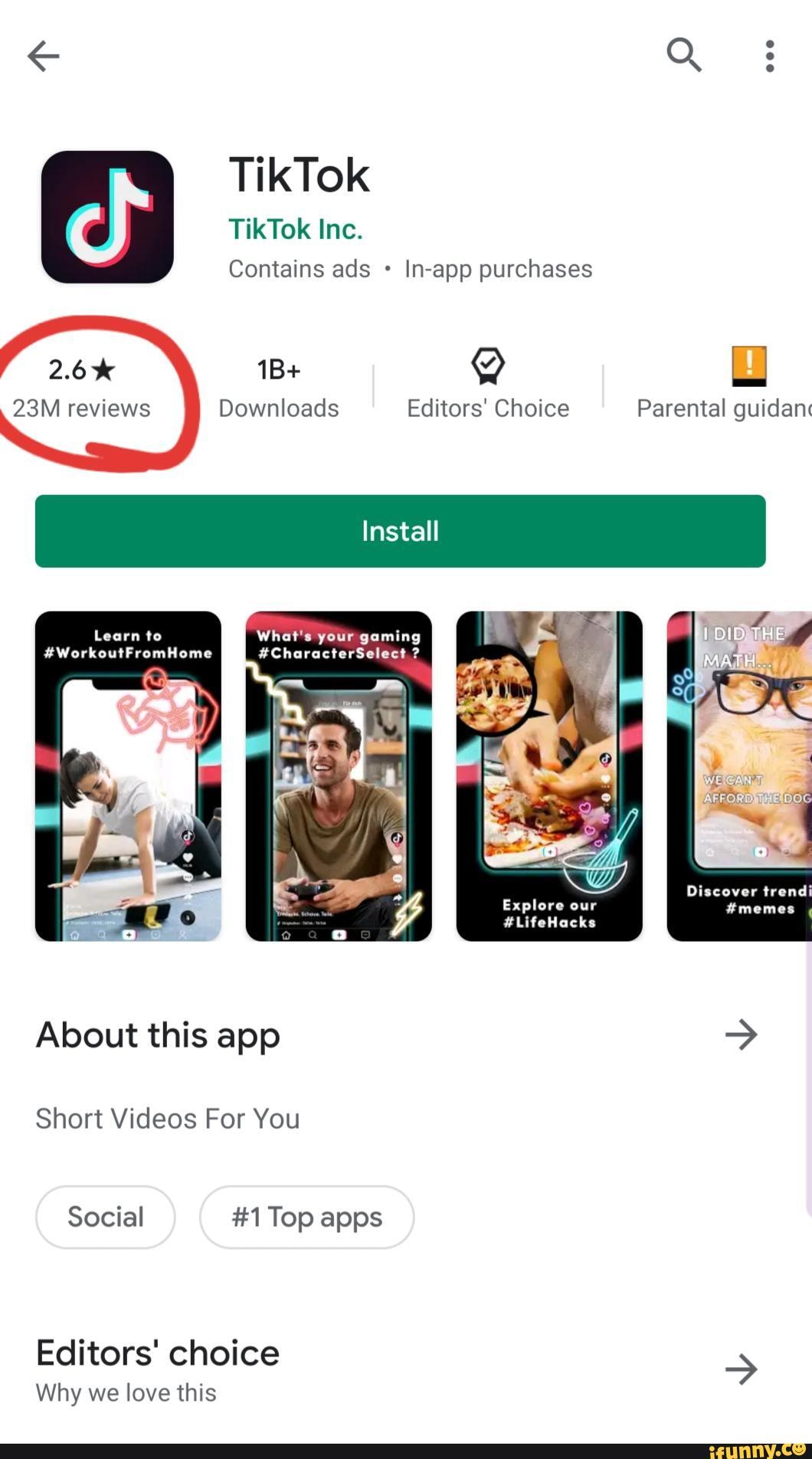This is a highly detailed screenshot from the Google Play Store, captured on a mobile phone or tablet. At the very top of the screen, there is a small left-facing arrow on the far left side, flanked by a magnifying glass icon for search, and three vertically aligned dots for additional options on the far right. Below this toolbar, the focus is on the TikTok app.

The TikTok module starts with its distinctive logo on the left side, followed by the app's name "TikTok" in bold black text. Underneath, in smaller green font, it reads "TikTok Inc." Further down, the text indicates that the app contains ads and offers in-app purchases. 

Prominently highlighted in a hand-drawn red circle are the app's ratings and reviews. TikTok has garnered a rating of 2.6 stars based on 23 million reviews. It also boasts over 1 billion downloads and is marked as an "Editor's Choice" app. There is a parental guidance warning included as well.

Below these details, a large, dark green "Install" button appears, with the text in white, inviting users to download the app. Further down, the screen offers a glimpse of various TikTok features through several screenshots illustrating potential posts. The screenshots include captions like "Learn to work out from home," "Watch your gaming character selection," "Explore our life hacks," and "Discover trends, memes."

Additionally, there's a section titled "About this app," highlighting that TikTok offers short videos for its users and is classified under social applications. Accompanying this is an "Editor's Choice" badge with a heading "Why we love this."